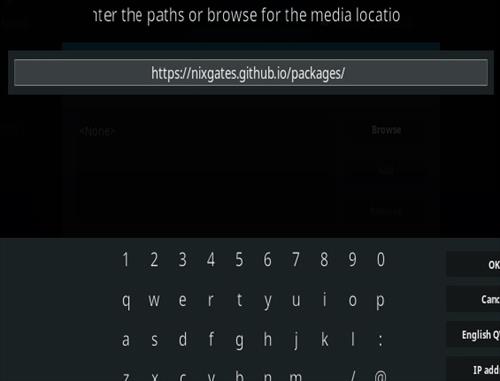The image depicts a digital interface that resembles a configuration page with a black background and grey text. At the top of the page, there is an instruction reading "Enter the paths or browse the media location," followed by a grey text box containing a URL link: https://nixgates.github.io/packages/. Below this text box is an on-screen digital keyboard, commonly found on tablets or mobile devices. The keyboard layout includes the number row from 1 to 0 and the typical QWERTY configuration: the first row consisting of the letters Q, W, E, R, T, Y, U, I, O, P, the second row of A, S, D, F, G, H, J, K, L, and a colon. There are also additional buttons on the side in black, which appear to include "OK" and "Cancel" options. The page seems designed for inputting or editing a webpage or media location, with references to an IP address suggesting connectivity or network configuration functionalities.